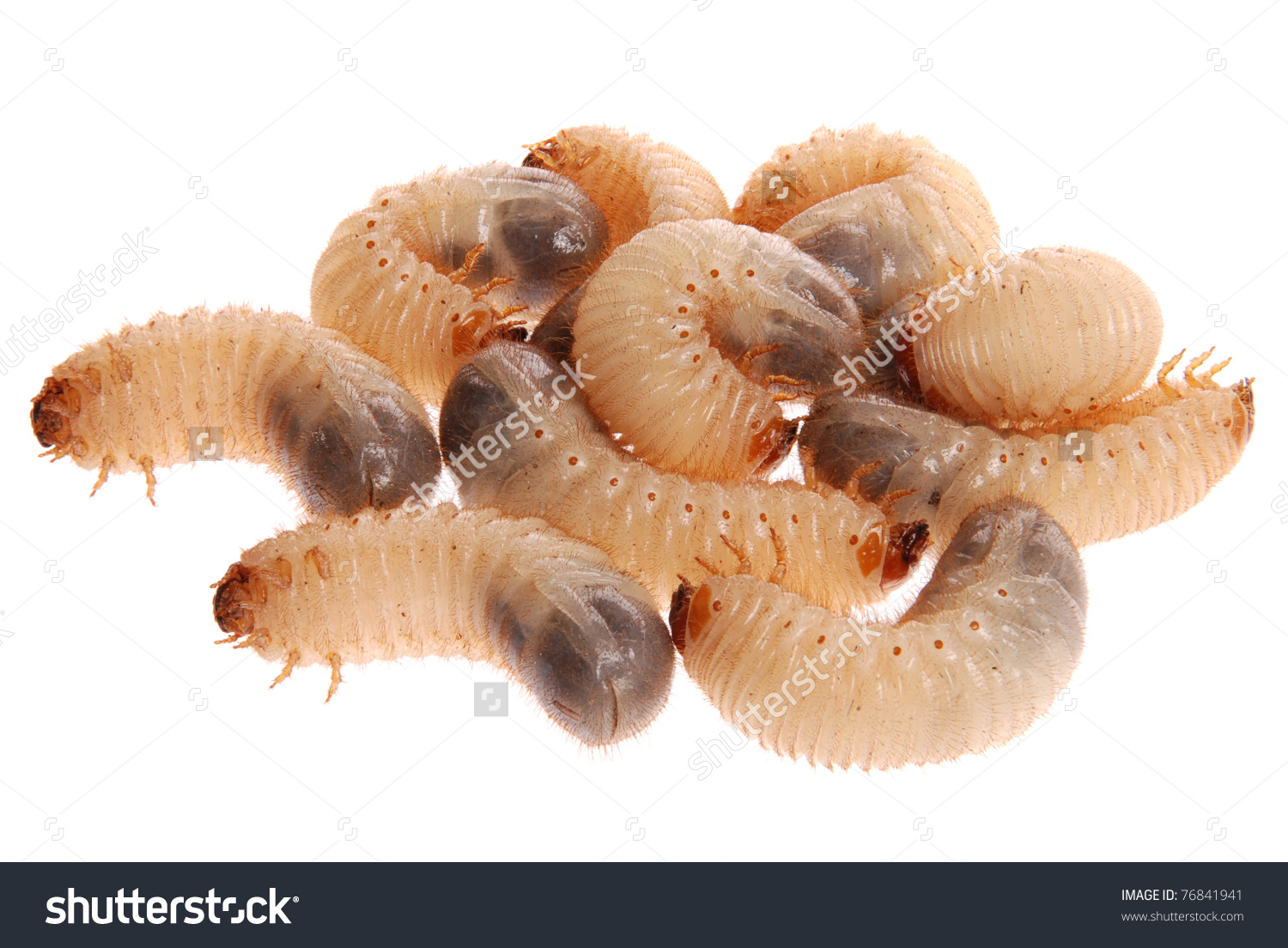The image depicts a group of approximately a dozen larvae or caterpillars, all gathered closely together on a white background. These insects are characterized by their fleshy, pink bodies adorned with red dots along their sides. They also feature very tiny, thin legs near their dark-colored heads, which contrast with their beige-toned middle sections. The ends of their bodies are darker brown. While some larvae appear curled up, others seem to be in motion, creating a dynamic scene. The background showcases a diamond pattern with light gray dashed lines, interspersed with the word "Shutterstock" appearing multiple times. At the bottom of the image, the text "shutterstock" is printed prominently across the larvae, with the left side noting "Image ID: 76841941" and a URL to Shutterstock's website.